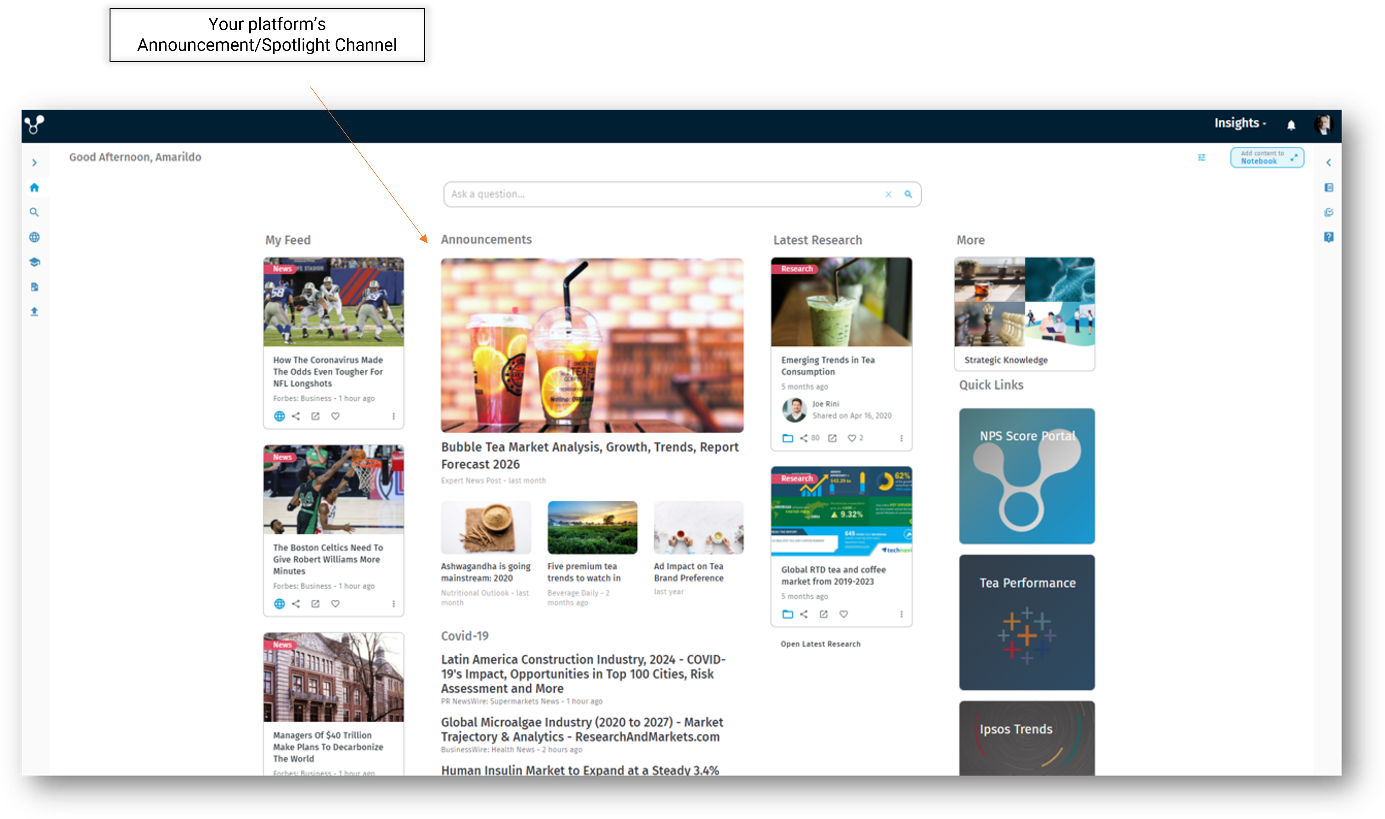The image depicts a website interface featuring a navy blue navigation panel at the top. On the left side of this panel is a small icon, while the right side includes options for "Insights," a notification bell, and what appears to be a login button. The main content area is divided into several sections:

- **My Feed:** This section displays a series of smaller-profile pictures.
- **Announcements:** Centrally located and highlighted by an orange arrow with the text "Your platform's announcement spotlight channel." This area is the focal point of the website, with larger, attention-grabbing images.
- **Latest Research:** Positioned to the right of the Announcements section, featuring images similar in size to those in My Feed.
- **More:** Another section with pictures comparable in size to those in Latest Research and My Feed.

The layout emphasizes the Announcements section as the primary visual element, supported by smaller, yet relevant, sections for My Feed, Latest Research, and More.